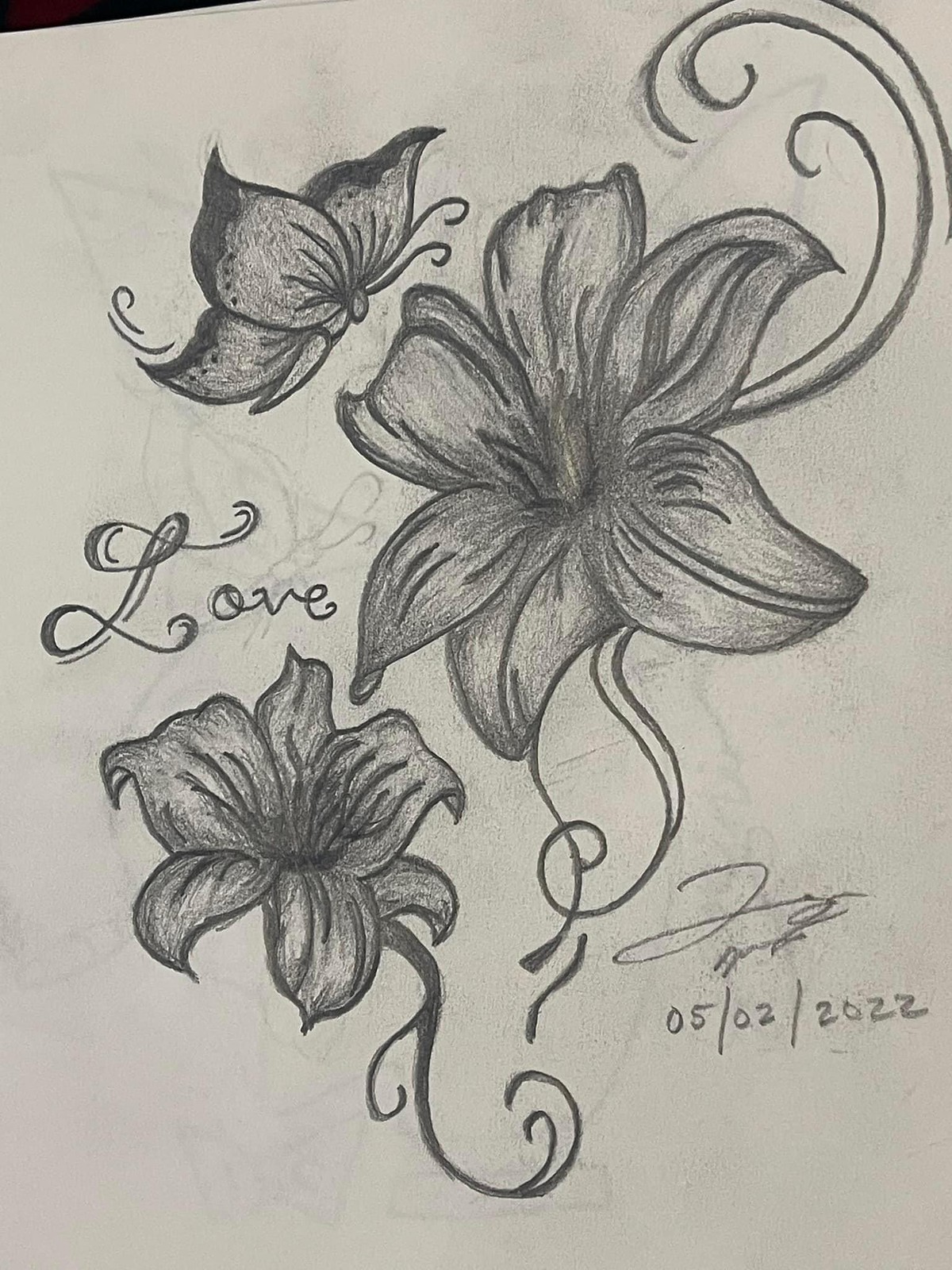This detailed graphite drawing, captured in a photograph, showcases two intricately designed lily flowers adorned with whimsical, swirling details representing their leaves and stalks. In the top left corner, a butterfly is gracefully approaching the larger blossom, adding a touch of natural elegance to the composition. Just below this enchanting scene, the word "love" is artistically scripted in flowing handwriting, further enhancing the drawing's romantic theme. In the bottom right corner, the artist's signature is prominently displayed, accompanied by the date "05/02/2022," marking the completion of this exquisite piece. Though the drawing is monochromatic, subtle hints of erased preliminary sketches faintly linger beneath the refined final lines, offering a glimpse into the creative process behind this captivating artwork.